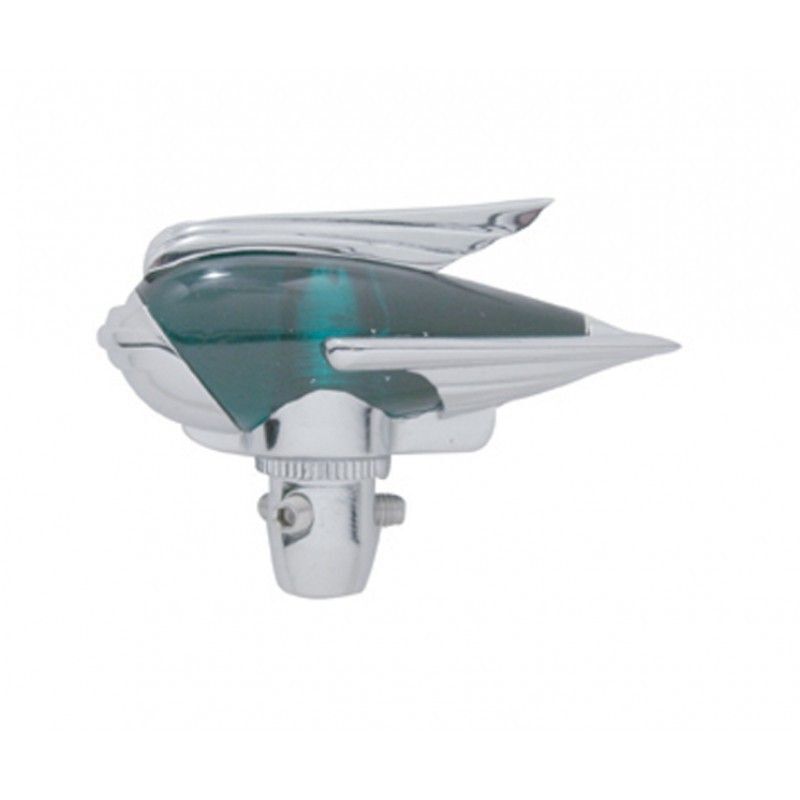The image features a peculiar object with a combination of silver-gray and turquoise-blue materials. The object appears to have a distinctive cylindrical bottom, possibly with four small prongs or extensions, and a neck area that includes a bolt and a washer. The top section is characterized by two pointed ends, covered by a translucent or plastic blue shield, which also has a molded connection to the gray parts. Lines or ridges are visible on the gray sections. Although its exact purpose is unclear, the object could be part of a motor, blender, or perhaps a device meant for an aquarium, and it features a wheel-like mechanism that might allow for adjustment or turning. No text or writing is visible on the object, adding to its enigmatic appearance.